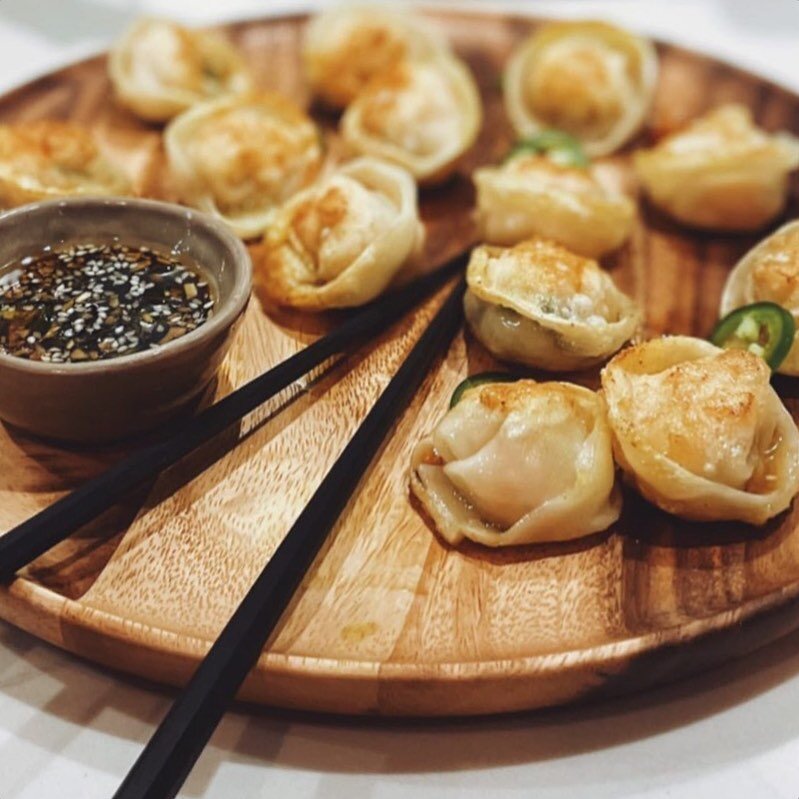The image depicts a delectable assortment of about a dozen golden-brown, fried dumplings, possibly chicken wontons or Japanese appetizers, arranged on a round, wooden serving platter. Each dumpling is garnished with a sliver of fresh green jalapeño, adding a vibrant touch of color. A small, round dish filled with a rich, dark soy sauce, speckled with sesame seeds and finely chopped seasonings, sits on the platter, inviting diners to dip and savor each bite. In the bottom left, a pair of sleek black chopsticks is poised, ready for use. The background subtly out of focus creates a slight depth, ensuring the dumplings are the central focus of the picture.